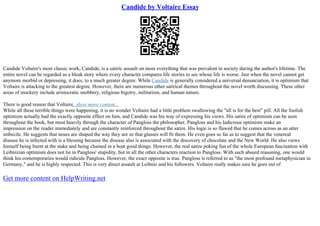The image is a screen capture of a document featuring extremely fine print, nearly blurred and illegible, set against a white background with black text. At the top, there is blue, underlined writing that appears to be a hyperlink reading "Candide by Voltaire Essay." Directly beneath this hyperlink is a black QR code. Below the QR code are two paragraphs of densely packed text estimated to contain approximately 1,600 words or more, though the exact content is unreadable due to the small font size. At the bottom left corner of the document, there is another blue hyperlink with the text "Get more content on helpwriting.net," suggesting additional resources. The overall appearance is indicative of screen-captured fine print, with no additional colors beyond the black and blue text on a white background.